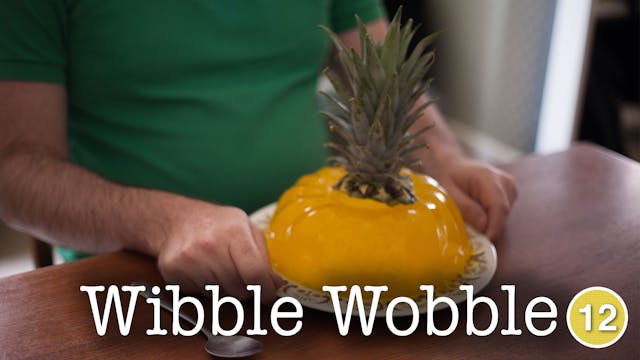In the photograph, a man wearing a green shirt and whose white, hairy arms are visible, is seated at a brown wooden table. He is holding a white plate with an ornate design around its rim. On the plate rests a yellow jello mold shaped like a bundt cake, with the spiny top of a pineapple placed directly in the center, giving the impression that the jello is pineapple-flavored. The image is set indoors, and the man’s head and legs are not visible. At the bottom of the image, the text "Wibble Wobble" is written in white lettering, and to the right of this, a yellow circle contains the number "12" in white text.